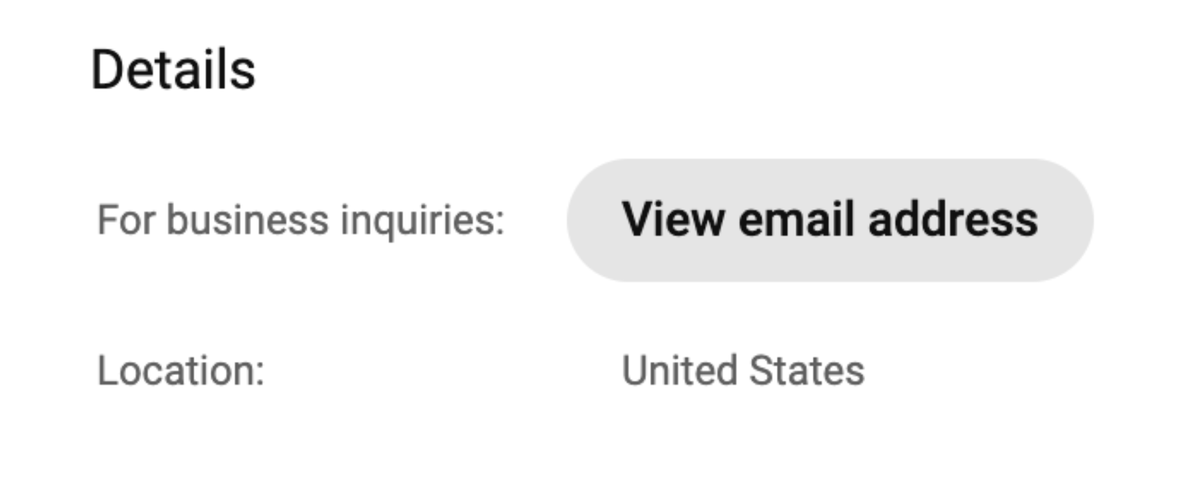The image is a close-up screenshot of a section from an application or website. At the very top left corner, the text "Details" is prominently displayed in black font. Below this heading, there is a subheading reading "For business inquiries." On the right side of the image, there is a gray button with the label "View email address" written in black text. Directly beneath this button, on the left side of the image, the word "Location" can be seen. To the right of "Location" and still under the "View email address" button, the text "United States" is displayed, indicating the geographical location information provided on this section.